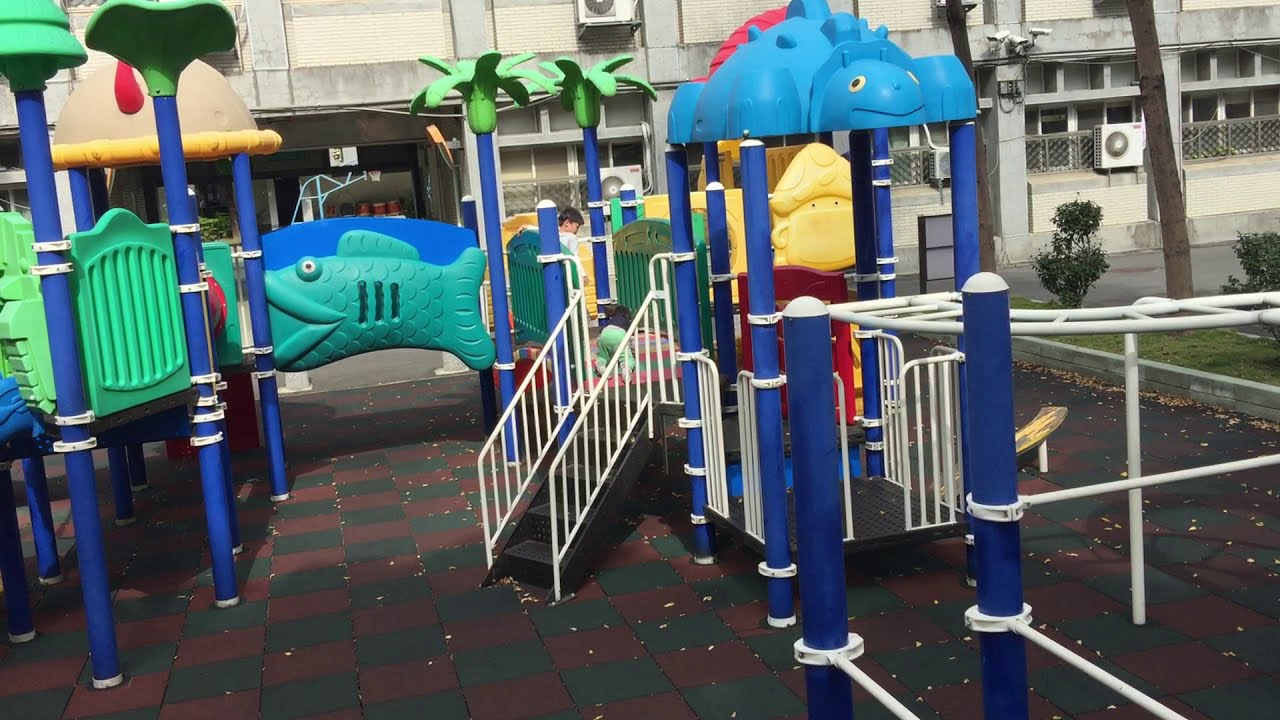This image shows an outdoor children's playground situated on a red and dark green tiled surface arranged in a checkerboard pattern. The playground itself is a vibrant and imaginative space featuring several play structures with blue poles. These poles are topped with caricatured representations of palm trees, their tops painted in shades of aqua and light green. 

Dominating the center is a jungle gym, decorated with various animal designs. A turquoise fish with white eyes and darker turquoise vertical stripes is painted on a blue background board. Its mouth is positioned near a blue pole on the left, and its tail touches another blue pole nearby. A yellow and tan dome can be seen over two of the blue legs on the left, adorned with something red hanging down. Another peculiar structure, resembling a yellow face with eyes and a hat, stands below and behind a blue turtle on four legs, part of the same playground setup.

Two young children are just barely visible, navigating the black steps of the labyrinthine play area. In the backdrop, a gray building with industrial elements like ventilation fans, air conditioning units, and conduit pipes adds an urban feel to the scene. There are partial fence-like coverings in front of some lower windows of the building. Some trees and grass are visible to the right, providing a touch of nature amidst the playful and industrial setting.